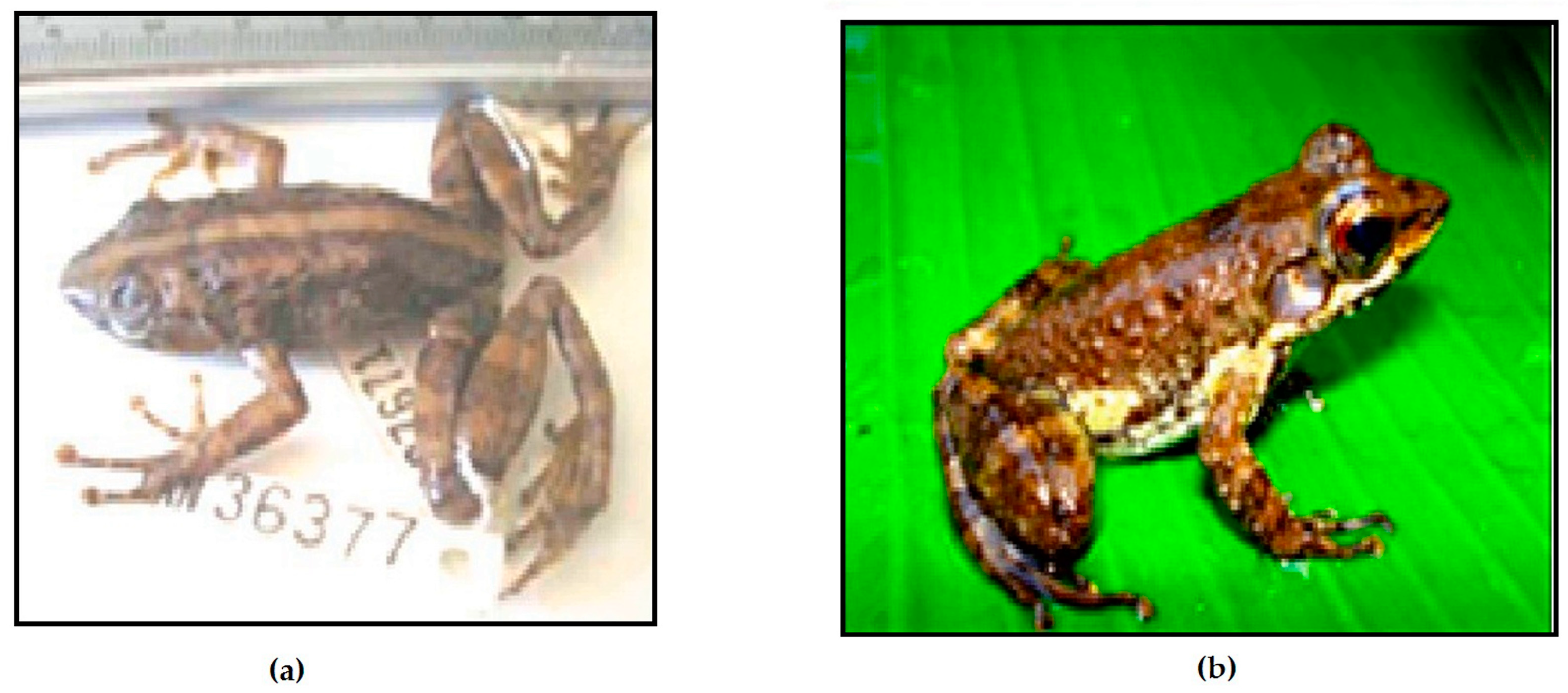The image features two distinct side-by-side photographs, each with a black border and labeled A and B respectively. In the left photograph (A), there's a brown frog with a prominent tan stripe running down its center and additional stripes on its legs. Its body is positioned flat against a white background, with a ruler at the top measuring its length. A printed number, 36377, appears at the bottom. Although it's uncertain whether the frog is alive, it seems to be part of a scientific context, perhaps an experiment or a study. The right photograph (B) shows a similar brown frog with a white chest but no central stripe on its back. This frog is vividly alive, perched in a classic crouching pose on a bright, light green leaf, with visible leaf veins running vertically. The frog in this image is facing right, contrasting with the left-facing frog in photograph A.